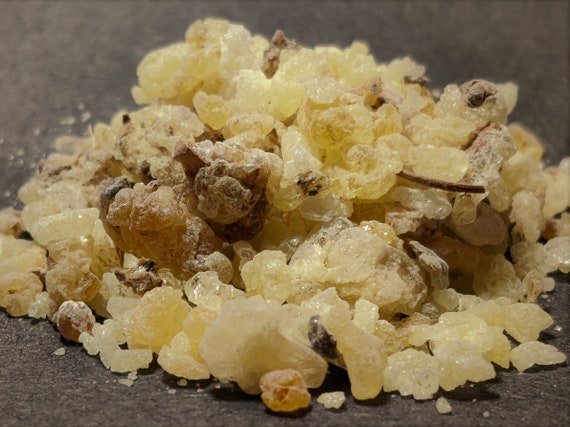The image depicts a collection of small crystal-type rocks scattered across a dark grey surface, likely resembling a table. These rocks appear primarily in shades of brown, transitioning from dark to light, and include tones of yellow and tan. The assortment is varied, with some rocks presenting a dull, opaque appearance while others gleam with clarity, exhibiting their crystal nature. Amongst the jumble, a twig is visible, suggesting the rocks may have been recently gathered. The pieces range in size from larger clumps to tiny specks and chips, some of which seem poised to break off from the main formations. The overall arrangement lacks any text, highlighting the intricate and multifaceted nature of the crystal rocks against the backdrop.